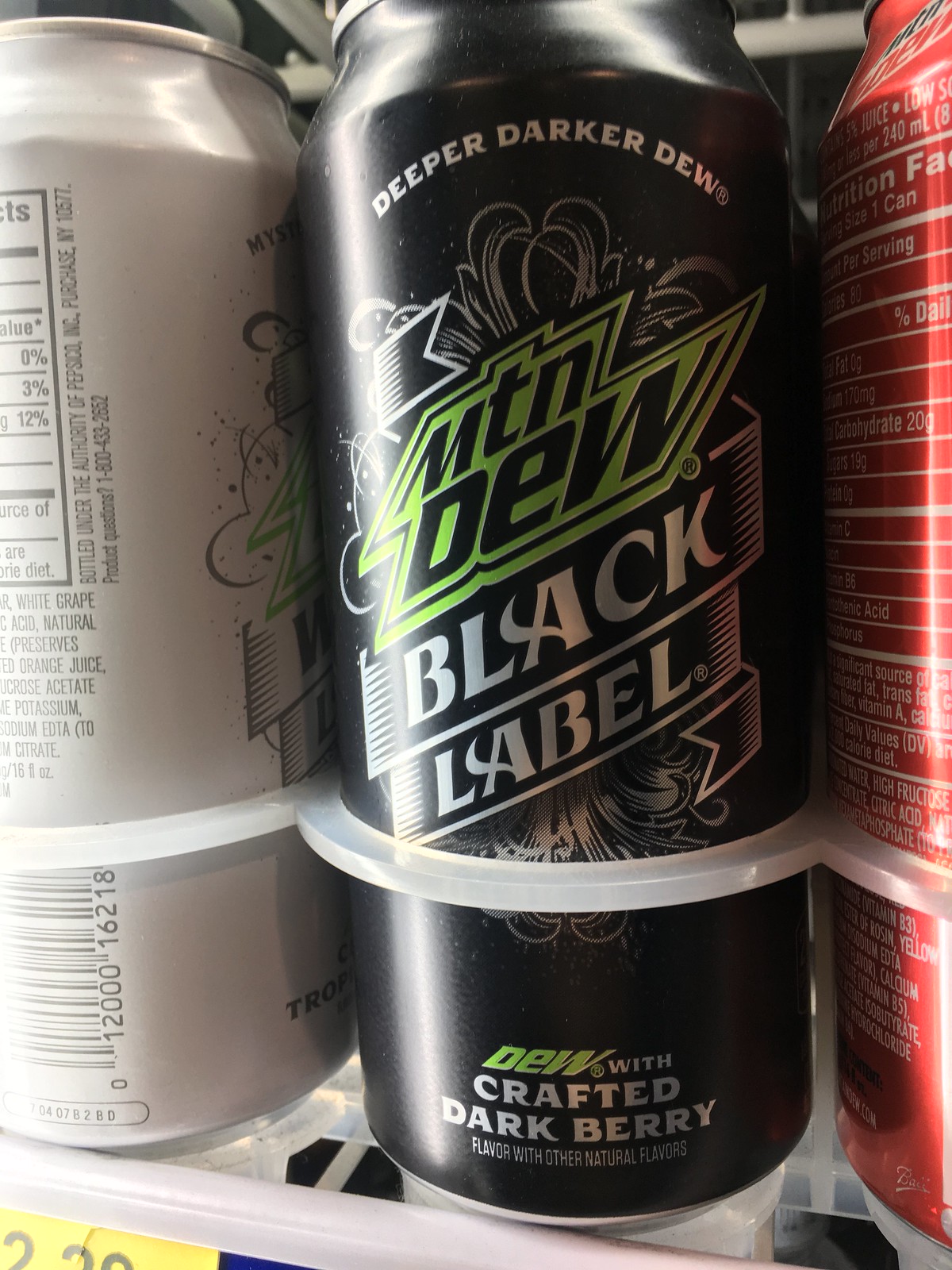This close-up photograph showcases three beverages displayed in a store, securely placed within a holder. The central focus is a tall, black can labeled "Mountain Dew Black Label." The can features elegant, vertical typography with the slogan "Deeper, Darker Dew" prominently displayed at the top in curved, white lettering. Below that, the can is detailed with the phrases "Dew with Crafted Darkberry" and "flavored with other natural flavors." The label is adorned with intricate crests or flares at both the top and bottom, adding to its sophisticated design.

To the left of the black can is a similar-sized white can, also bearing the Mountain Dew branding. While only the side of this can is visible, one can make out a comparable logo design. At the bottom edge, part of the word "tropical" is discernible, hinting at the flavor. Additionally, portions of the nutrition label, ingredient list, and a side view of the barcode are partially visible.

On the right-hand side, there is a red can, again of a similar size to the others. Visibility is limited, but the top section where the can tapers inward reveals a faint Mountain Dew logo. The nutrition facts are printed in white text. The details beyond this are obscured, making it difficult to discern additional information about this particular can.

The photograph captures the intricate details and varied design elements of these Mountain Dew products, emphasizing the branding and packaging aesthetics.